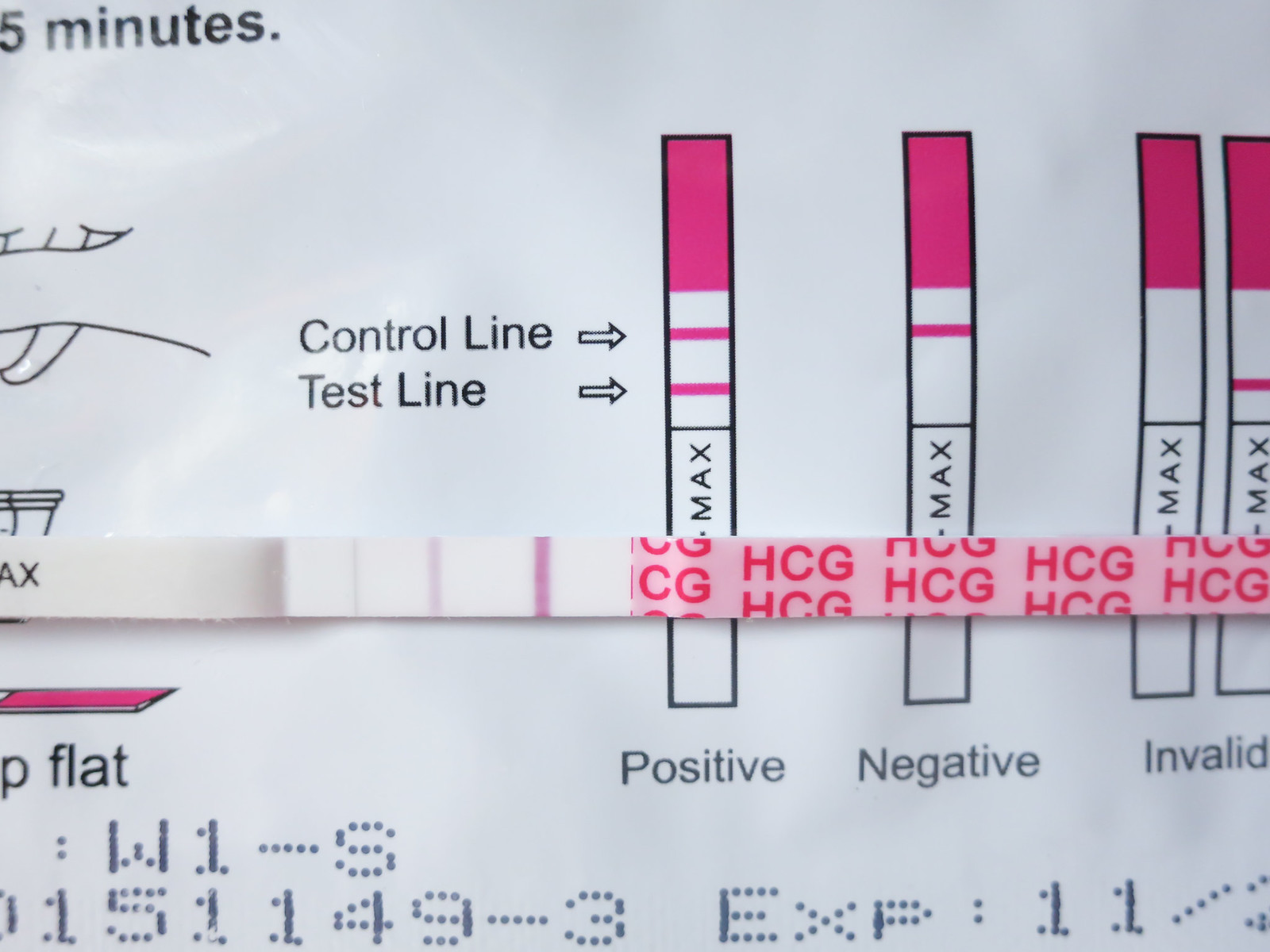This image depicts a completed urine test displayed on a white piece of paper. The test strip features a clear and distinct control line as well as a test line, which indicates a positive result. The strip itself is predominantly white, marked with the letters "AX" on the left side. Along the strip, there are two pink stripes followed by a pink-colored section. The test is designed to detect the hormone HCG (human chorionic gonadotropin), indicated by the letters "CG" followed by "HCG".

The chart on the paper elucidates what different results mean: a positive result is shown by two lines, a negative result by one line, and an invalid result by no lines or any inconsistency in markings. At the top left corner of the paper, a timer notation indicates "5 minutes," providing a timeframe for the test outcome. The bottom part of the paper shows the expiration date, and beneath that, a code labeled "W1-S" followed by the serial number "151149-3."